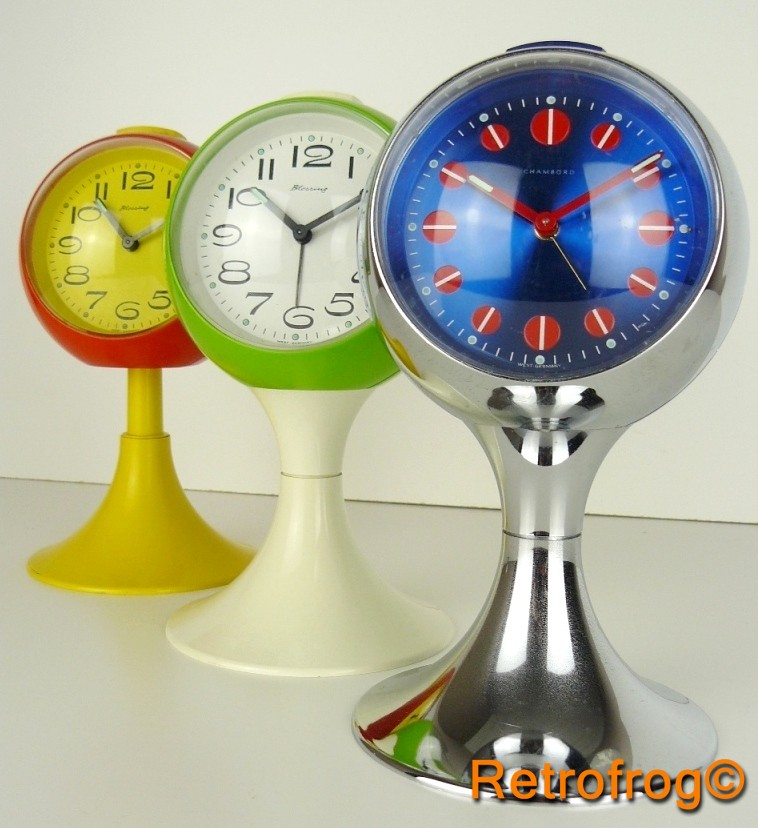The photograph depicts a charming collection of vintage-style clocks, each showcasing distinct mid-century modern design elements. Positioned on a pristine white counter with a white wall serving as the backdrop, these three clocks exude a nostalgic yet contemporary appeal.

The foremost clock features a striking silver-toned base, likely made of metal or plastic, which elegantly tapers at the center before flaring out again to support the clock's face. The dial, a bold cobalt blue, is adorned with vibrant red circles at the 12, 3, 6, and 9 o'clock positions, accompanied by smaller circles at the intervening hours. Each circle is accentuated with a white line, while minute markers are intricately positioned between them. The clock hands are a vivid red, tipped with white, adding a dynamic contrast against the cobalt backdrop.

Behind it, the second clock boasts a white base supporting a green body, maintaining the same graceful hourglass silhouette. Its face is a clean white, featuring stylized black numbers interspersed with minute tick marks. The black clock hands, complemented by the additional second hand, stand out prominently, offering clarity and simplicity.

The third and final clock in the collection diverges slightly with a cheerful yellow plastic base and stem, transitioning seamlessly into a red body. Its face is a warm yellow, housing black while silver hands. The numbers are rendered in a stylized black font, juxtaposed with minute tick marks that enhance readability.

Together, these clocks create a visually engaging display, merging retro aesthetics with contemporary design sensibilities.